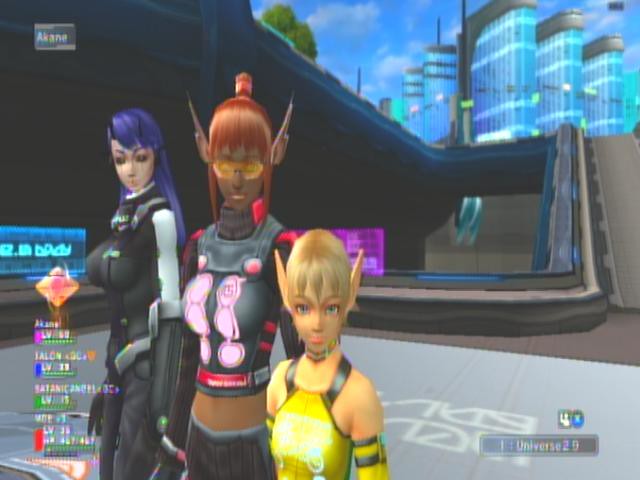This image is a detailed screenshot from a video game, featuring a group of three distinct characters standing in a row on a concrete floor against a backdrop of a cloudy sky and a turquoise-colored building with a greenish roof. To the left of the building, trees are visible, and a platform extends from the left side of the image, traverses under the buildings, and descends into a staircase on the right side. 

In the foreground, the three characters are arranged in a group photo style. On the left stands a woman with purple hair, wearing a black and gray uniform, possibly featuring black arm plates. The character in the middle has orange, auburn hair styled up in a small bun with some pieces hanging in the front, and she has elf-like ears. She wears a distinct black and red uniform with pink accents. To her right is a shorter character with blonde, very short hair, also with elf ears, dressed in a yellow and black uniform.

Additional game-related elements such as a health and status bar are visible on the left and lower right sides of the image.